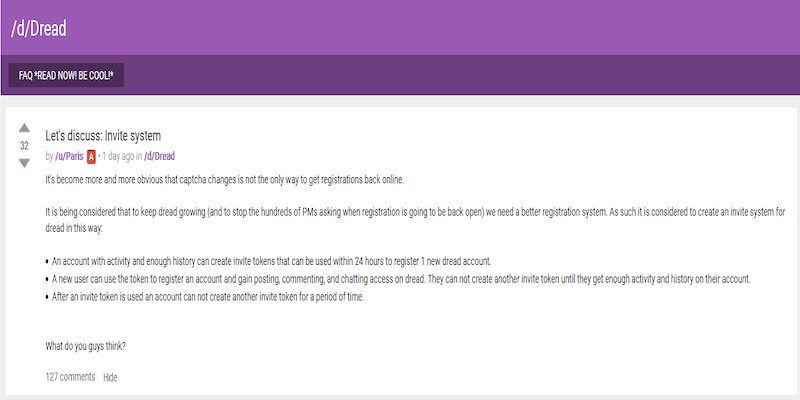The screenshot features a web page displayed in landscape orientation. At the top, a purple horizontal bar spans the width of the page, displaying white text that reads "\/D\/dread". Directly beneath it is a darker purple bar containing options such as "FAQ," "Read Now," and "Be Cool."

Below these bars, a headline introduces a social media post. To the left of the headline, there are up and down arrows likely representing voting or liking functionalities. The post includes a headline, a username accompanied by an icon, a timestamp of when it was posted, and the name of the forum it was posted in.

The main body of the post features a paragraph of text followed by three bulleted points, offering more details. At the bottom of the post, there's a prompt asking, "What do you guys think?" alongside the count of 127 comments and an option to hide the post.